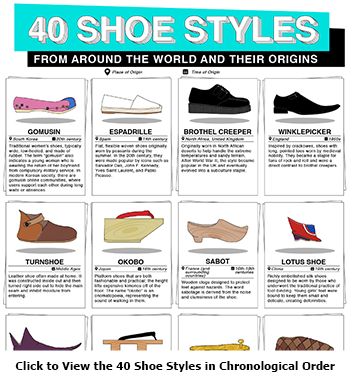The image is a vertical, rectangular infographic showcasing various shoe styles from around the world. At the top, there's a turquoise banner with the text "40 SHOE STYLES" in bold, white 3D letters. Beneath it, a black banner with white capital letters reads "FROM AROUND THE WORLD AND THEIR ORIGINS." The image features cartoon-like illustrations of shoes arranged in three rows, although the third row is partially cut off. Each shoe illustration includes a title and a brief description. In the first row, from left to right, are: 'GOMUSIN,' a pink flat shoe with a blue top; 'ESPADRILLE,' a white casual shoe; 'BROTHEL CREEPER,' a larger black shoe; and 'WINKLE PICKER,' a low-cut pointy black boot. The second row includes: 'TURN SHOE,' a brown moccasin-like shoe; 'OKOBO,' a wooden platform thong sandal; 'SABOT,' a wooden clog; and 'LOTUS SHOE,' a red and blue shoe. Each shoe is depicted in its traditional colors with a gray shadow underneath. At the bottom of the image, text in black font instructs viewers to "click to view the 40 shoe styles in chronological order."